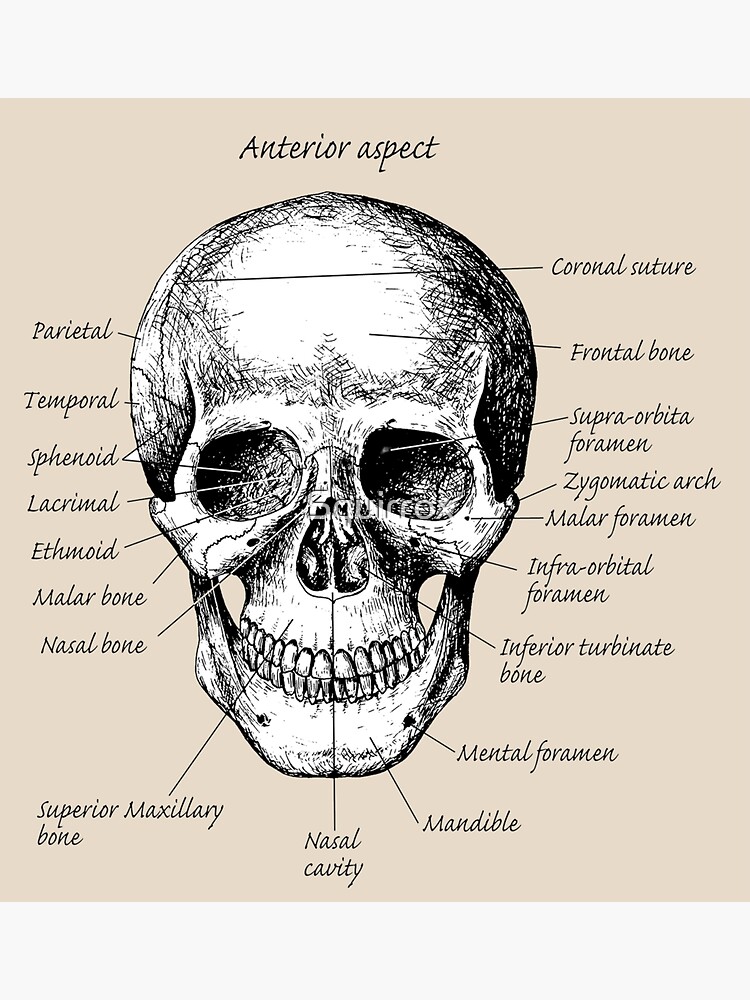The image depicts a detailed, black-and-white illustration of a human skull, rendered in a style that employs scratch shading. The skull faces forward, against a light tan background, and features numerous anatomical labels in black text. 

At the top of the skull, the label "Anterior Aspect" is prominently displayed. On the right side, annotations include "Coronal Suture," pointing to the top of the skull; "Frontal Bone," indicating the forehead; and "Supraorbital Foramen," marking the bridge of the nose. Further down, labels such as "Zygomatic Arch" (above the ear), "Malar Foramen" (under the eye), "Infraorbital Foramen" (center of the eye), and "Inferior Turbinate Bone" (below the nasal passages) are noted. Towards the chin, the "Mental Foramen" and "Mandible" are specified.

The left side annotations start with "Parietal" at the top, followed sequentially by "Temporal," "Sphenoid," "Lacrimal" (indicating the tear ducts), "Ethmoid," "Malar Bone," "Nasal Bone" (pointing to the nose), and "Superior Maxillary Bone."

The image also features a watermark, which appears to read "Sauirrox." The combination of anatomical precision and artistic detailing makes this illustration both informative and visually engaging.